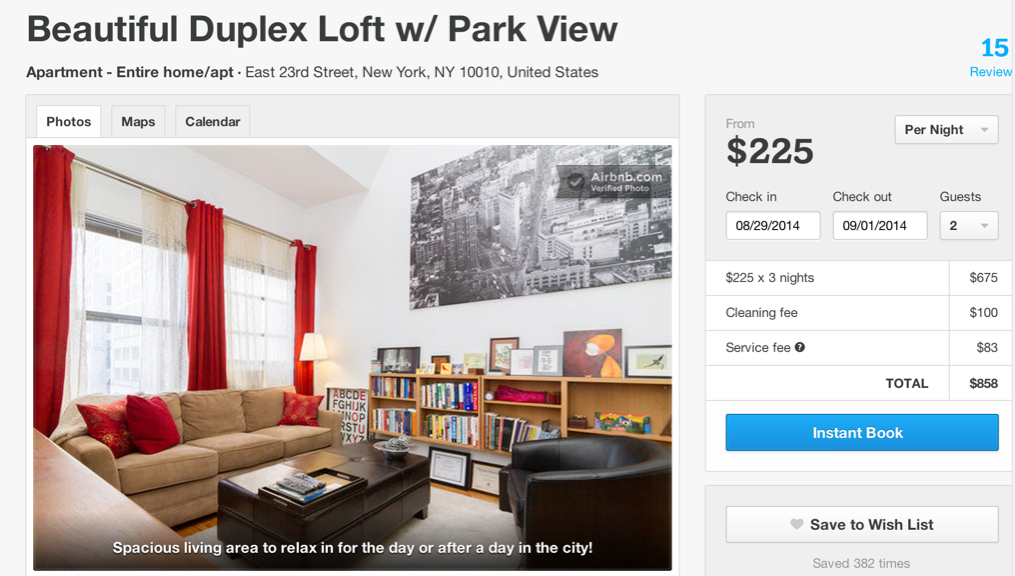A website screenshot showcases an apartment available for nightly rental. At the top, the page prominently advertises a "Beautiful Duplex Loft with Park View." The property is listed as an "Apartment, Entire Home/Apartment" located at East 20th Street, New York, NY, 10010, USA. 

Below this title are tabs for "Photos," "Maps," and "Calendar," with "Photos" being highlighted. The image displayed focuses on the living area of the apartment. The left side of the picture features a window adorned with curtains, while the right side showcases a wall with a cityscape picture. A bookcase lines the wall beneath the picture, and a comfortable couch is positioned in front of the window. There is also an additional chair in the room. The overlay text on the photo reads, "Spacious living area to relax in for the day or after a day in the city."

To the right of the image is detailed information about the property, including a nightly rate starting at $225. The example booking details provided are for a check-in date of 08-29-2014 and a check-out date of 09-01-2014, accommodating two guests. The cost breakdown displays $225 multiplied by three nights, totaling $675, with additional fees including a $100 cleaning fee and an $83 service fee, bringing the total to $858. There are interactive buttons labeled "Instant Book" and "Save to Wish List." The property has been saved 382 times by users.